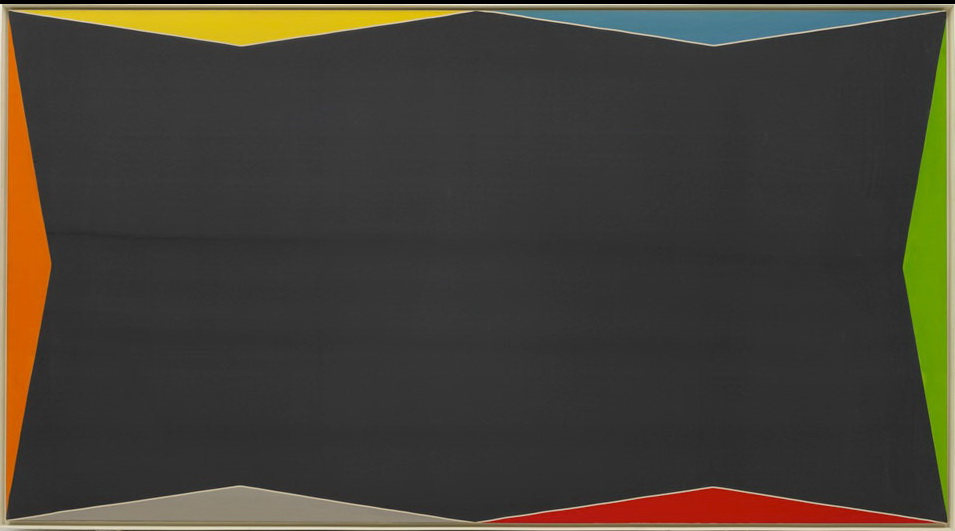This digital artwork features a horizontally aligned rectangular image predominantly filled with a solid black background, bordered by a thin silver line. Geometric shapes, specifically colorful triangles, are arranged symmetrically around the interior of the rectangle, forming a striking border. At the top, two wide-based triangles, one yellow and one blue, are positioned upside down. The left side of the rectangle is accented by an orange triangle with its tip pointing towards the right, while the right side features a green triangle with its tip pointing towards the left. The bottom edge is adorned with two upright triangles, a gray one on the left and a red one on the right, completing the geometric frame. These vibrant shapes, set against the stark black background, are the primary focus of the image, creating a dynamic and visually engaging composition.